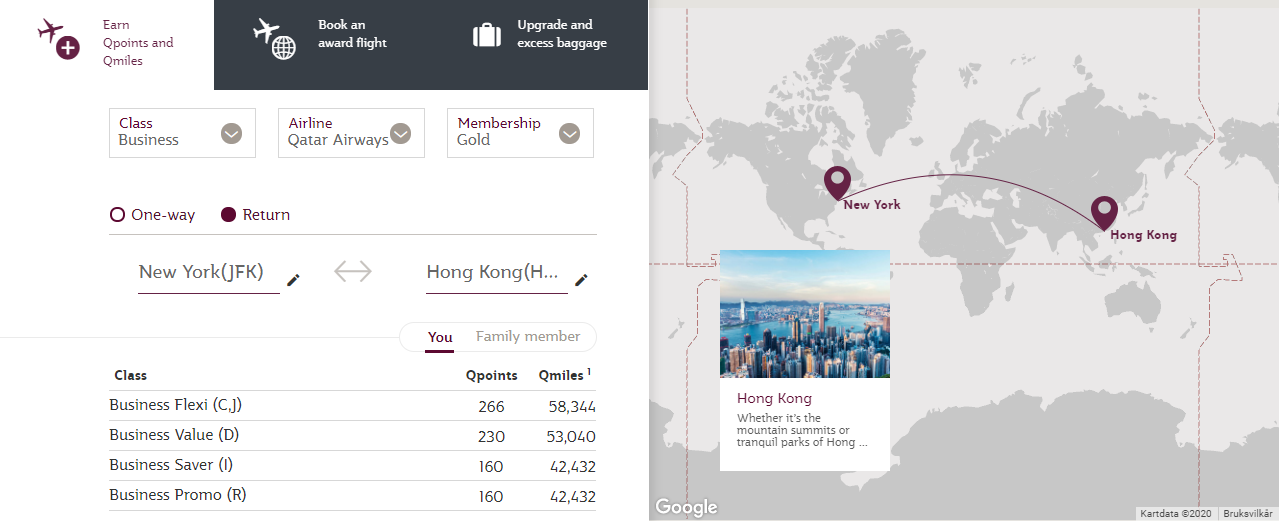Side by side images provide detailed insights into a flight itinerary and its related map. On the left, the flight information is presented with an assortment of burgundy icons and font at the top, featuring an airplane, a circle, and text that reads "Earn Q Points and Q Miles." Below, a black box with white icons displays an airplane and a globe, alongside the label "Book an Award Flight." Additionally, a suitcase icon indicates "Upgrade and Express Baggage."

Further down, a series of boxes with burgundy and silver text outline essential details: “Class: Business,” “Airline: Qatar Airways,” and “Membership: Gold.” Options for "One Way" and "Return," both in burgundy font and each accompanied by a circle, are also shown. The "Return" option is highlighted with a filled burgundy circle. The itinerary details "New York JFK" underlined with a pencil icon, followed by an arrow pointing to "Hong Kong," similarly underlined with a pencil icon and paired with a gray arrow.

A detailed chart breaks down various classes and mileage options. The “Class Business Flexi” highlights 266 Q Points and 58,344 Q Miles, while “Business Value D” shows 230 Q Points and 53,040 Q Miles. Both “Business Saver” and “Business Promo” list 160 Q Points and 42,432 Q Miles.

On the right side, a gray map visually connects New York to Hong Kong using a burgundy arrow with points marking the path. An accompanying image showcases downtown Hong Kong under a clear blue sky, featuring striking skyscrapers. The text in purplish-burgundy font reads "Hong Kong," followed by a partially cut-off description: "Whether it's the mountain summits or tranquil parts of Hong Kong." A copyright mark at the bottom indicates the year "2020" accompanied by the Google watermark.

This detailed depiction not only provides comprehensive flight details but also visually enhances the travel experience from New York to Hong Kong.